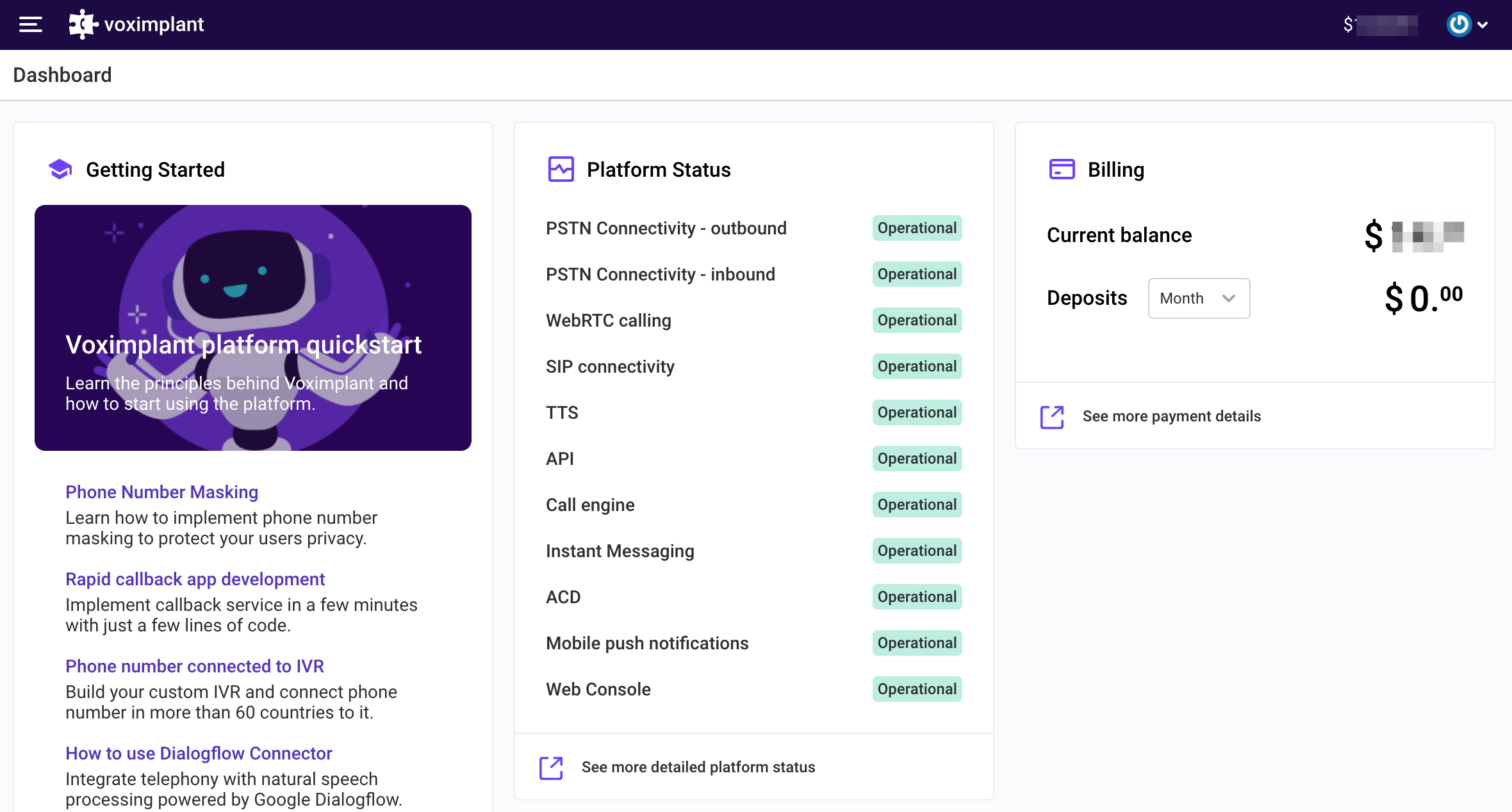In the screenshot of a computer interface displayed with a light gray background, a purple rectangular bar spans the top of the page. On the left side of this bar, three horizontal lines resembling a menu icon are visible next to a small white logo. The text "Vox Implant" marks the webpage's identity. In the upper right corner of the purple bar, there is a dollar sign followed by an empty rectangle, alongside an icon and a downward-facing arrow.

Beneath this header, the page is divided into three distinct columns. The left column, labeled "Getting Started," features a purple icon next to it and includes a square image depicting an alien character set against a purple background. This section contains four statements, each beginning with a purple heading followed by explanatory text in black.

The central column, titled "Platform Status," also begins with a purple icon. Below this title, a list of status indicators with descriptive words is displayed. Each status indicator on the right side of this column is marked with a green rectangle labeled "Operational."

On the rightmost side of the screen is the "Billing" column. Here, sections labeled "Current Balance" and "Deposits" are present, though the balance information is obfuscated, shown grayed out and blurred.